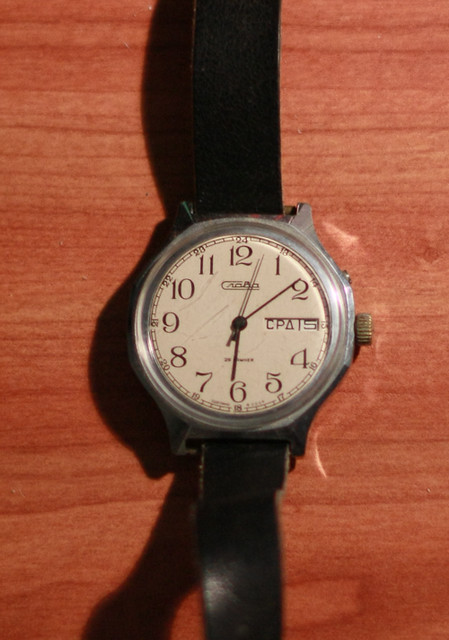In this photograph, we observe a vintage wristwatch elegantly displayed on a wood grain table, likely stained in a deep mahogany hue. The watch is positioned vertically with its narrow, black leather straps running straight, framing the centerpiece of the composition. The watch face, large and circular, features block-style numbers and is slightly discolored, hinting at its age. Marking the time at 6:08, the watch displays a precise arrangement of hour, minute, and second hands, with the second hand poised between the 12 and 1. Adding to its vintage charm, there is an inscription "CPA5" on the face, along with a rusted winding mechanism on its side. The watch’s exterior is secured by small silver screws, further emphasizing its antiquated craftsmanship. The overall image captures not just the timepiece, but a sense of history and nostalgia.